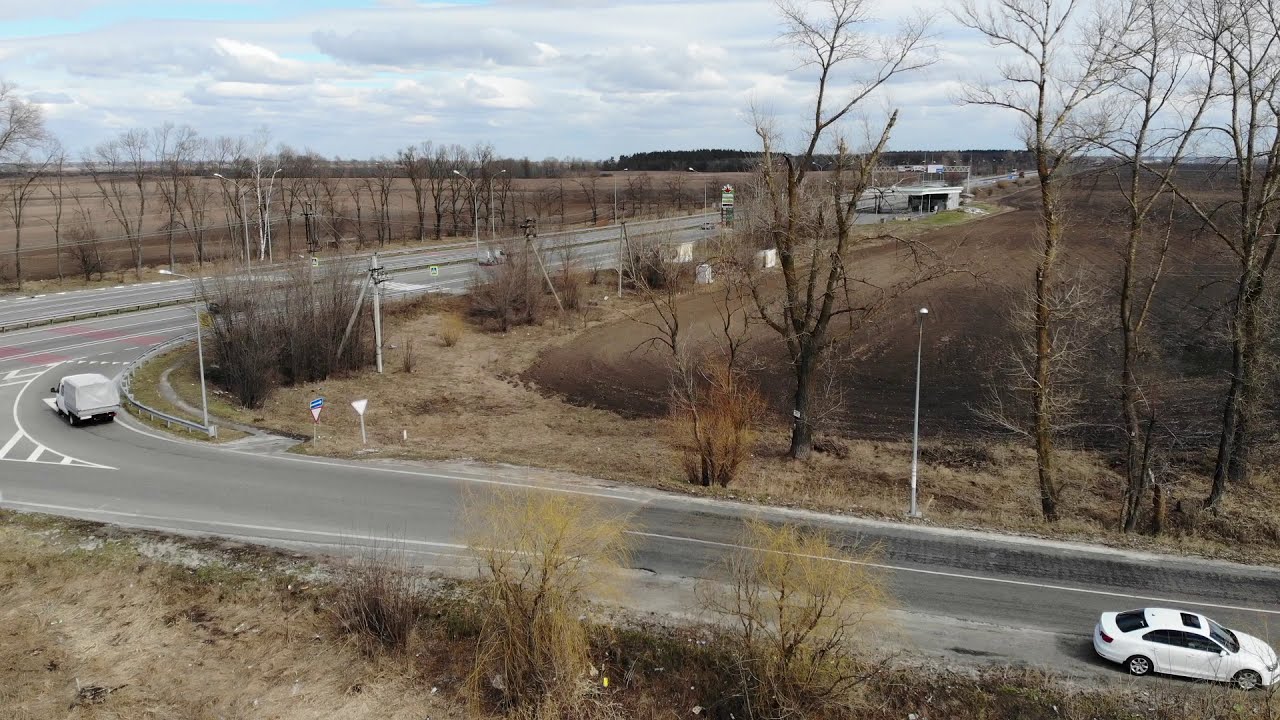The image depicts a barren autumn landscape centered around a freeway. The scene shows a two-lane road beginning at the bottom right corner, intersecting and merging into a larger, multi-lane highway that curves off into the horizon toward the top right. The sky is light blue with patches of white clouds. The environment is desolate, characterized by brown earth and an array of dead, leafless trees. A white sedan is visible at the bottom right, driving toward the edge of the frame. Further along the road, at the point where it converges with the highway, a white van makes its turn. The highway itself is expansive, featuring several lanes divided by a grassy median. Sparse traffic populates the road, and there are few structures, with only a faint, black-and-white structure possibly indicating a distant gas station or convenience store. Lampposts line the road, enhancing the sense of emptiness and desolation in the overall scene.